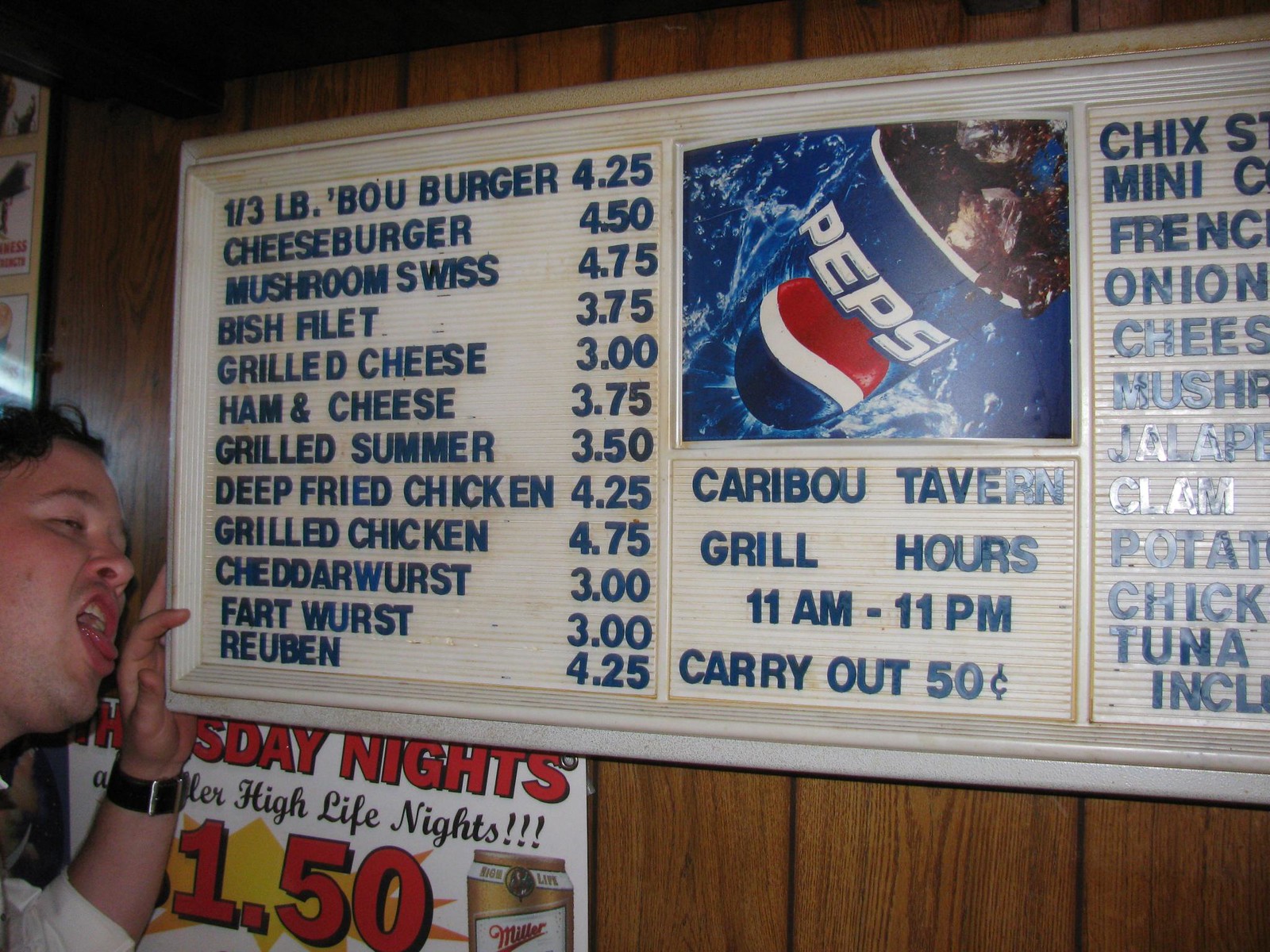A person is standing at the bottom left corner of the image, playfully holding a large, vintage-looking white menu mounted on a brown-paneled wall. The person is making a quirky face at the menu. Below the menu, partially obscured by the person’s hand, is a Miller High Life beer advertisement, stating "Wednesday nights" and "High Life Nights $1.50" alongside an image of a beer can. The menu itself is divided into three panels, with a Pepsi bottle prominently displayed at the top middle panel. Below the bottle, the words "Caribou Tavern" are visible along with the grill hours: "11 a.m. to 11 p.m." and a note about a 50-cent carry-out charge. The left panel features a detailed list of menu items with prices, including: Third-pound Boo Burger for $4.25, Cheeseburger for $4.50, Mushroom Swiss for $4.75, Fish Filet for $3.75, Grilled Cheese for $3.00, Ham and Cheese for $3.75, Grilled Summer for $3.50, Deep-Fried Chicken for $4.25, Grilled Chicken for $4.75, Cheddar Wurst for $3.00, Fart Wurst for $3.00, and Reuben for $4.25. The right part of the sign remains partially out of the image frame.